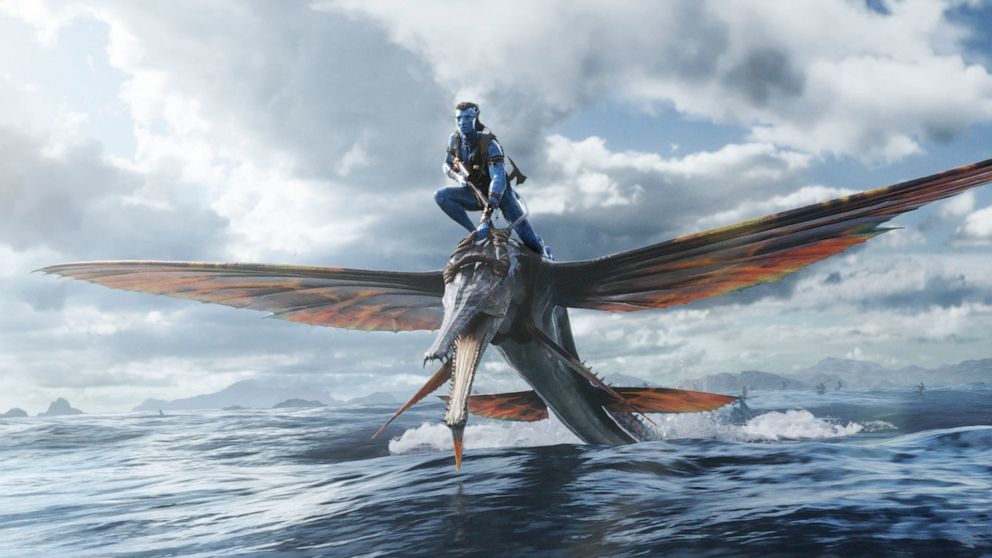In this animated, rectangular illustration, we see a dramatic scene set against a cloudy, predominantly dark sky. Emerging from a large body of water, possibly an ocean, is a fearsome, bird-like aquatic creature. This monster, reminiscent of a dragon, features a long, crocodile-like beak revealing sharp, jagged teeth. Its sleek, scaled body has large, sweeping wings extending from its back, with smaller wings near the tail, giving it a formidable and fantastical appearance.

Perched on top of the creature’s head is a blue-skinned figure, evoking images of an Avatar character, dressed in black combat gear. The figure, crouching low, holds a gun in his right hand, which is braced against his knee. Additionally, a hatchet is visible, tucked into his belt. The water below shows ripples and waves, emphasizing the creature’s movement as it rises. The background extends into a distant mountain horizon, shrouded by thick clouds that cover 60% of the sky, with a hint of sunlight piercing through from the top left corner. This image, rich with detail, feels like a vivid scene from a high-fantasy video game or movie.